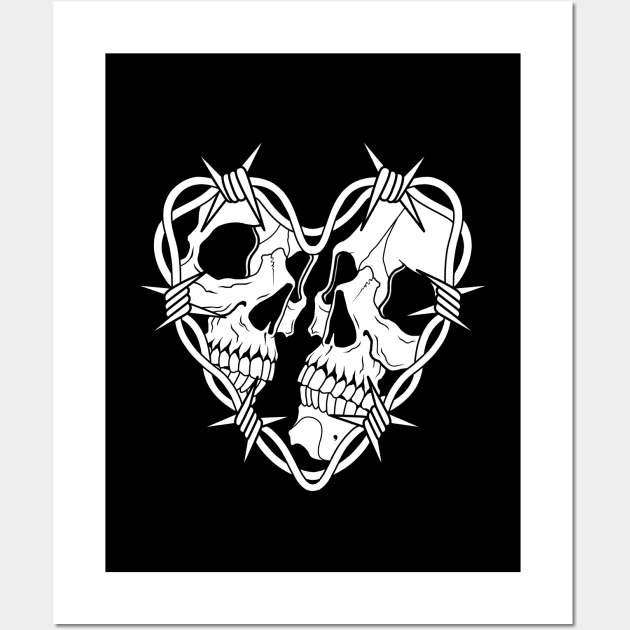The image depicts a black-and-white artwork featuring two skulls, facing each other, encompassed by a heart-shaped outline formed from barbed wire. The background is solid black, enhancing the stark monochrome contrast. The left skull is smaller, aligned in height with the larger right skull, but positioned slightly higher. Both skulls have finely detailed teeth—approximately 16-17 in the larger skull and 12-13 in the smaller one—with their mouths almost touching. The barbed wire heart surrounding the skulls features six distinct coils, each resembling barbed wire points. A notable detail includes a small black dot near the chin of the right skull. The entire composition has a minimalist yet detailed quality, evoking a sense of undying love, and is suggestive of tattoo or comic book art styles.